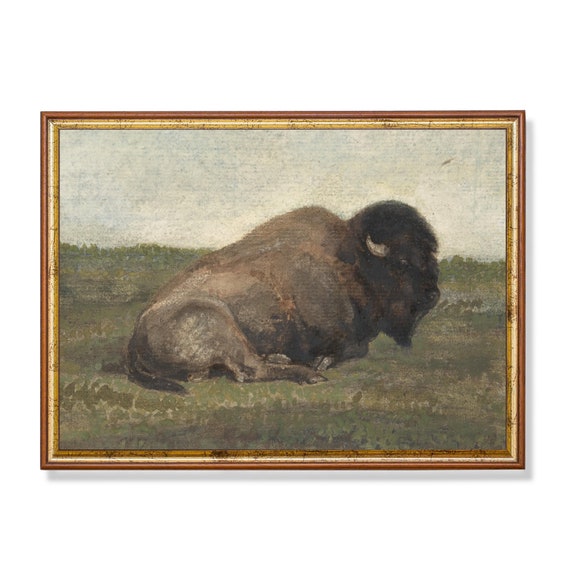This is a vintage style painting of a full-grown American buffalo sitting calmly on a grassy plain, framed by an intricate brown and gold frame. The buffalo, with its distinctive large head of black fur, showcases a pair of white horns and has a dark, almost black, nose and eye visible. Its fur gradually transitions from dark brown at the front to a lighter shade towards the rear, with a medium-length tail matching the dark hue of its head. The animal’s muscular back legs are tucked underneath it as it sits on the dull green grass. The background features a muted blue sky with hints of white, suggesting the presence of clouds. The overall palette consists of calm, muted colors, creating a serene and detailed piece reminiscent of classic artwork often seen in museums or as a distinguished centerpiece on a wall.